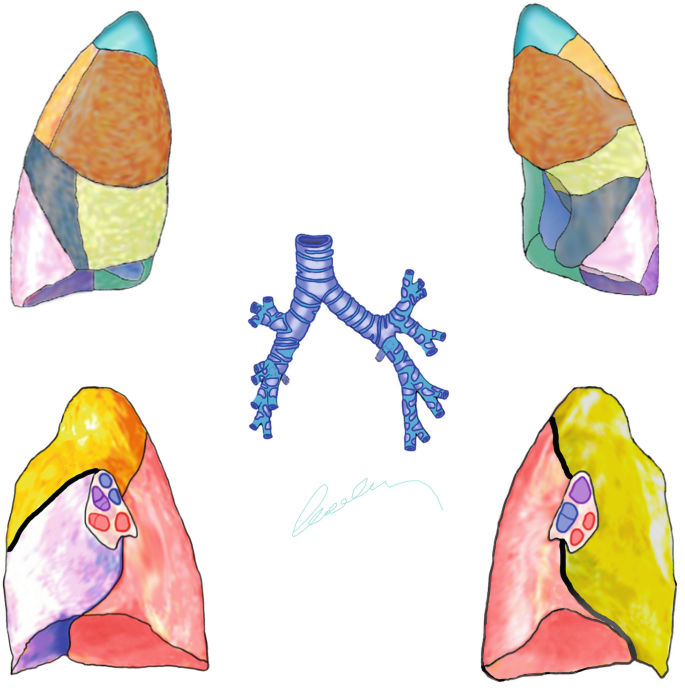The image is an educational, color-coded, almost animated illustration depicting the lungs and trachea from various angles, likely intended for medical instruction. At the center, the trachea is prominently displayed in light blue with darker blue veins, branching into a thick tube that bifurcates into right and left sections, representing the main bronchial passages. Each branch further subdivides, illustrating the complex network of airways within the lungs. The trachea ends with multiple smaller tubes, highlighted in different colors to signify various lung functions.

On the top left and right are detailed drawings of the lungs' front view. The left lung is segmented into multiple colored sections indicating different lobes and their respective functions: light blue at the top, followed by brown, light purple, dark blue, grayish hues, and ending with a purple and green section. The right lung shows a similar color-coded pattern from top to bottom, with variations in shades and sections.

The bottom part of the image displays the lungs' posterior views. The left lung in this section features a golden top, transitioning to purple, pink, and darker purple colors, enhanced with intricate detailing of the lung's thickness and lobes. Adjacent to it, the right lung from the backside mirrors the golden, pink, and dark pink hues with a small white area containing blue and pink circles suggesting representations of specific lung features or functionalities.

This comprehensive illustration vividly covers the anatomical features of the lungs and trachea, utilizing a rich palette of colors to differentiate between the various lobes and their positions, making it an effective tool for understanding lung anatomy and functionality.